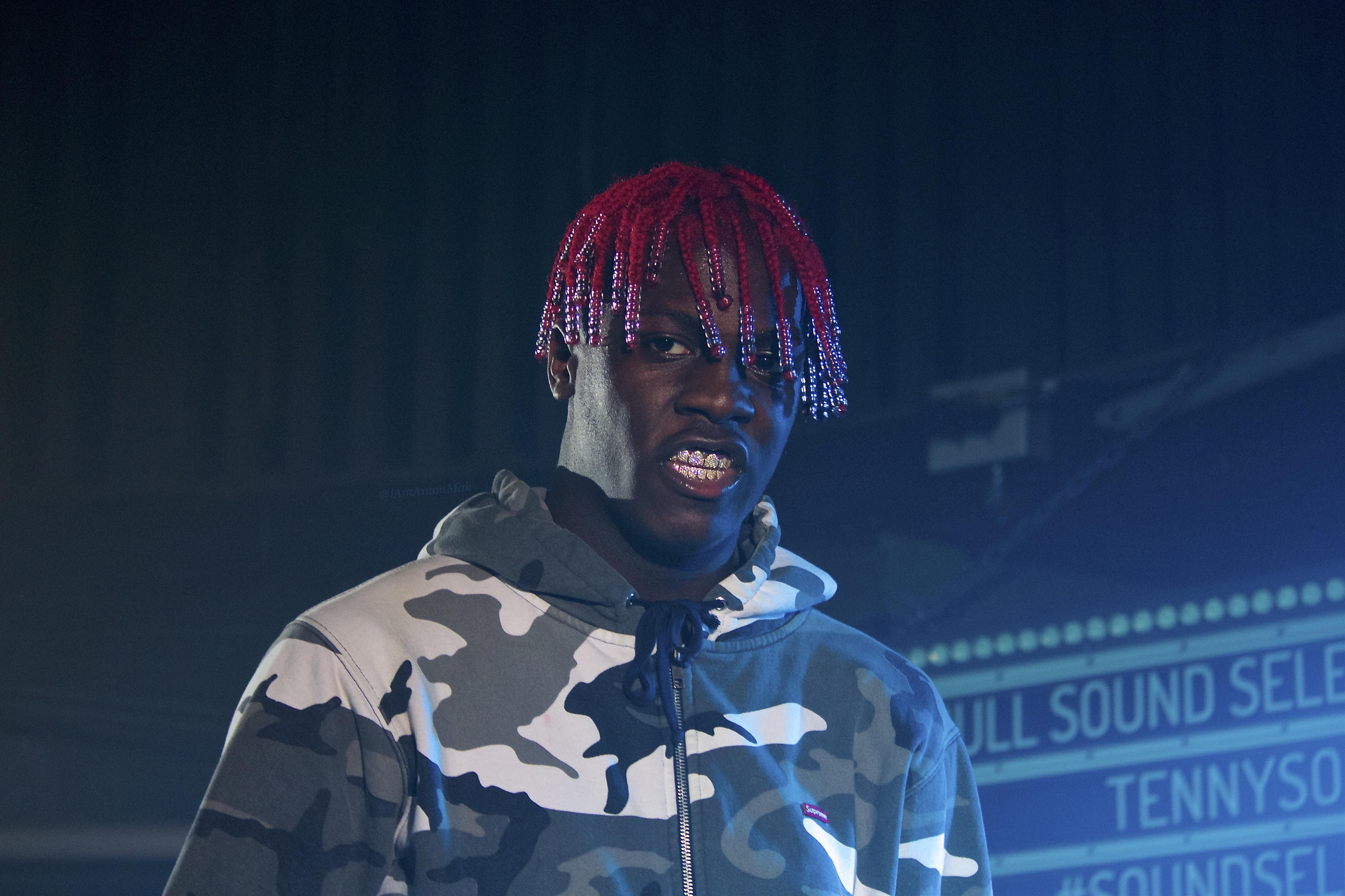In this photograph, an African-American man is positioned centrally, wearing a grey, black, and white camouflage-patterned jacket. His distinct red hair is fashioned into dreadlocks, each adorned with clear beads and a single red bead at the end. The dreadlocks hang long enough to partially cover his face. He has his mouth open in an oval shape, revealing his teeth, as if he is mid-sentence or possibly expressing emotion, but he is not smiling. The background is predominantly dark, suggesting an indoor setting with low lighting. On the right side of the image, there is a sign with white lettering. The visible portion of the sign reads "NOLA Sound System, Tony's Civilization," and includes the hashtag "Sound Selection." This setting and signage indicate he might be in a music venue.